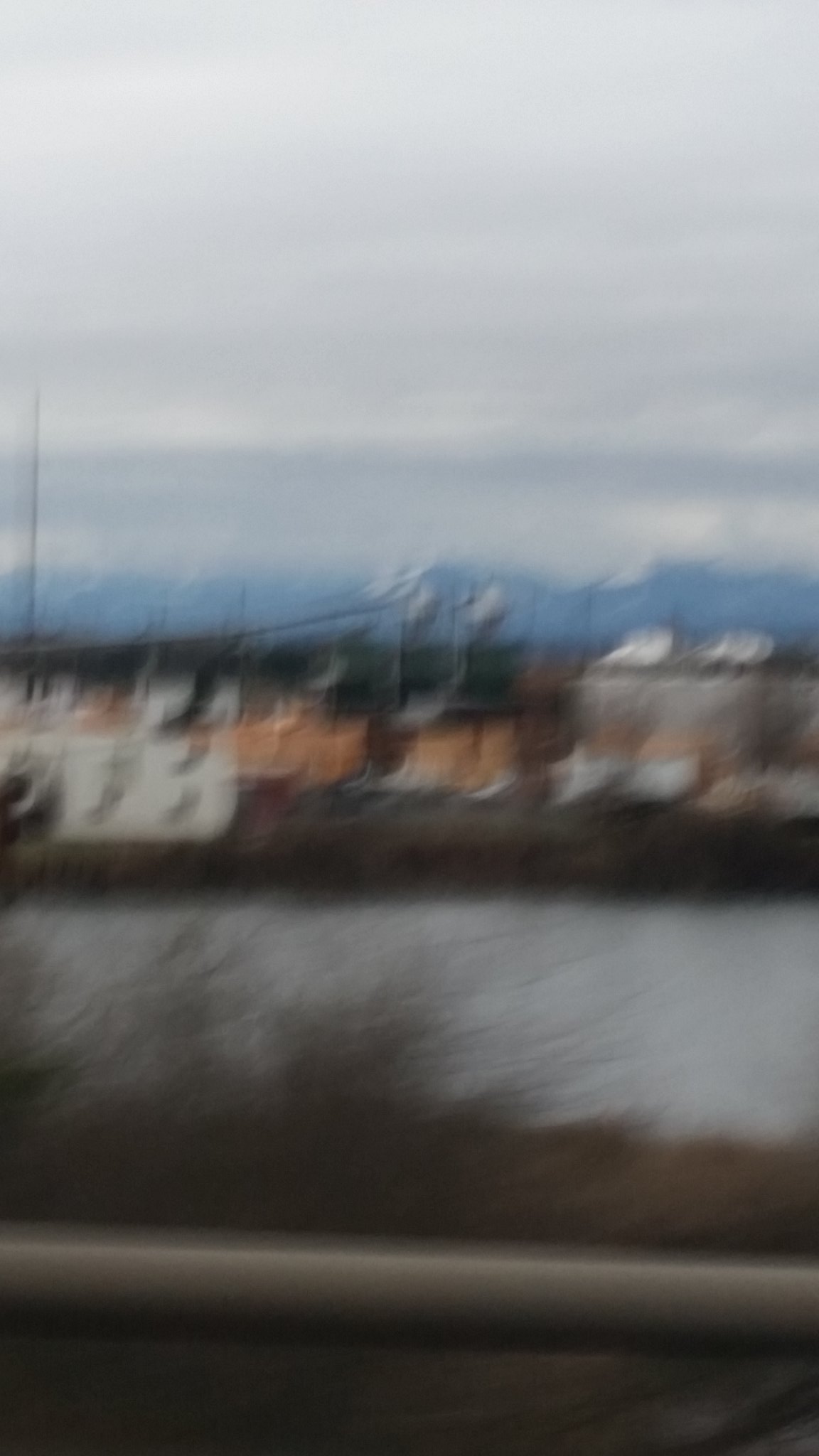A slightly out-of-focus image capturing a serene riverside with a blend of natural and urban elements. In the foreground, a metal cylinder railing runs along the bottom edge, leading into a patch of brown, withered grass. The river's surface, painted in shades of gray, stretches across the middle of the scene. On the far bank, a mixture of green and brown hues signals the earth, while a smattering of indistinct white, orange, and gray buildings forms a modest cityscape. Above, a slender strip of blue sky transitions into a canopy of gray clouds, completing this tranquil urban river view.